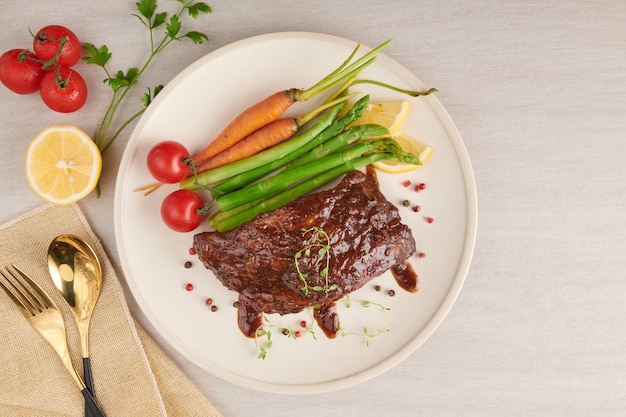A meticulously arranged bird's eye view image features a round white plate centered on a light grayish pink background. The plate holds a small rack of ribs generously lathered in dark brownish-red barbecue sauce, adorned with a few sprouts. Atop the ribs rest a couple of full, vibrant orange carrots and a few stalks of tender green asparagus. Two small red tomatoes on the vine sit comfortably on the right side of the plate, accompanied by two bright yellow lemon wedges. Scattered alongside are some red and black round seeds for added detail.

To the left of the plate, a tan cloth napkin is thoughtfully spread out, hosting a set of elegant silverware—a fork and spoon with golden tops and dark gray bases. Just above the silverware rests half a juicy lemon, cut to reveal the fleshy insides. Further to the left, three tomatoes cluster together still attached to their vine, adding a pop of color next to a sprig of cilantro that lends a fresh, green accent to the scene.